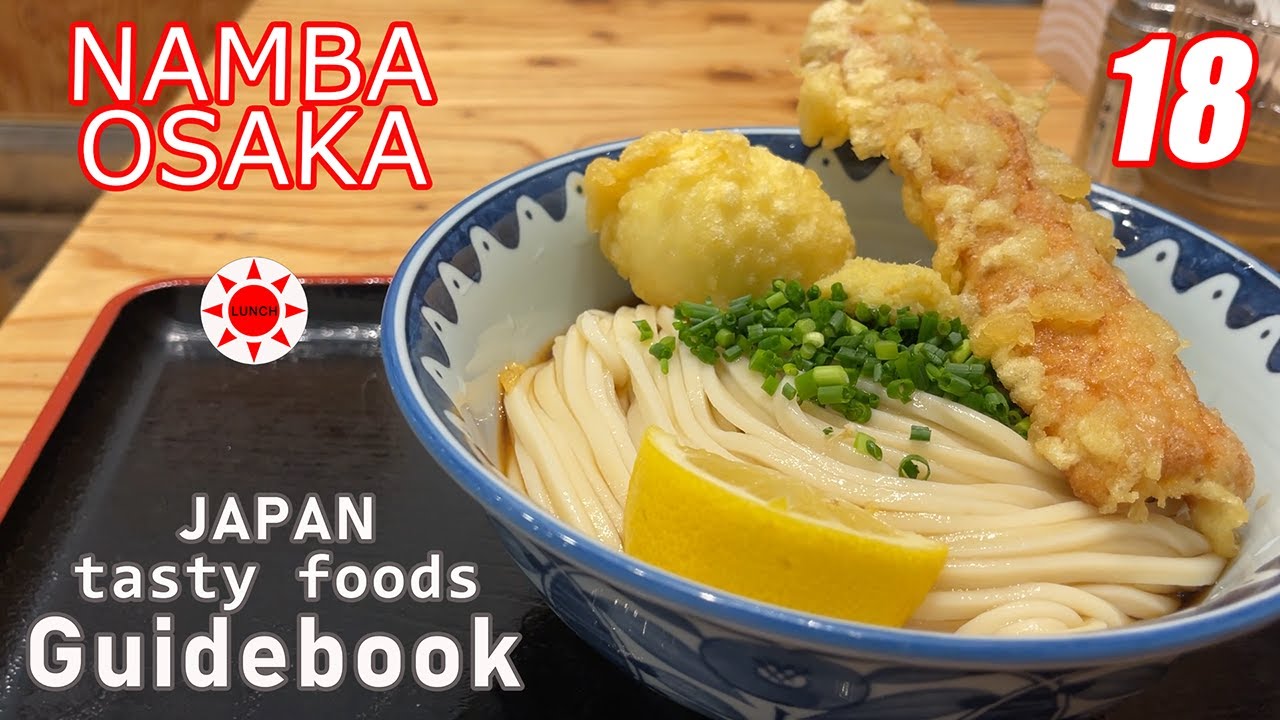The image showcases a vibrant and enticing portrayal of Japanese cuisine, specifically linked to Namba, Osaka, as indicated by the red and white text in the upper left corner. Dominating the scene is a large, detailed bowl that features a blue exterior and a white interior, highlighted with a blue rim around the edge. Inside this visually appealing bowl rests a bed of noodles, generously topped with finely chopped green onions or chives. Adding layers of texture and flavor, the bowl contains a fried dumpling and a piece of tempura, possibly vegetables, positioned on the right-hand side. A fresh lemon slice delicately accents the rim of the bowl. Below and to the side of the bowl, the text "Japan Tasty Foods Guidebook" invites viewers to discover the best culinary destinations in Japan, suggesting that this image could either grace the cover of a physical guidebook or serve as a vibrant introduction to a food-related video series. The number "18" in the upper right corner hints at categorization or sequencing within the guidebook or video series.